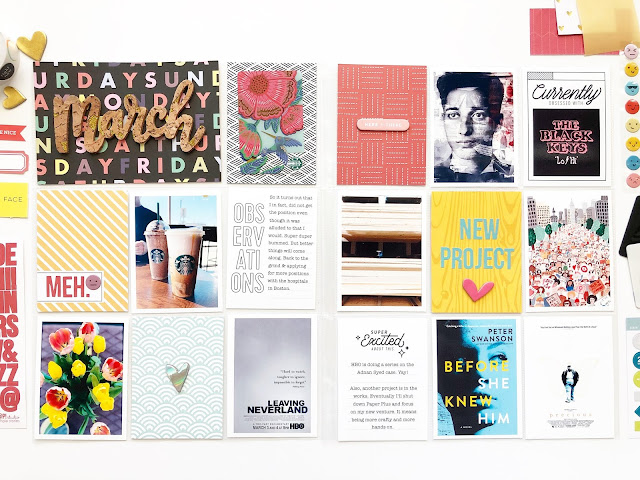The image depicts a collage of various cards and items, each with unique and distinct features. At the top, the word "March" is prominently displayed. Among the assortment is a card featuring a vibrant red dahlia with green leaves, set against a checkerboard background. Adjacent to it is a red card with a tongue depressor, designed to resemble a woven pattern.

A black and white photograph of a man draws the eye, with a striking smear of red on one side. Below this, a note reads "currently the Black Keys," potentially indicating a musical event or playlist. Next, an image resembling a scene from South Park showcases the iconic characters.

A piece of wood marked with "new project" and a checkmark introduces a sense of accomplishment. The next card shows separated mini blinds, revealing a dark night outside. Following this, the word "OBSERVATIONS" is partially spelled out, creating a sense of mystery.

Further along, the Starbucks logo is easily recognizable. A yellow and white striped pattern card adds a touch of brightness. A cheerful bouquet of tulips precedes a heart placed on silver wrapping paper, evoking feelings of warmth.

At the bottom, an advertisement for the HBO documentary "Leaving Neverland" grabs attention. A burst of excitement is conveyed with the phrase "Super excited." Concluding the collage is what appears to be a book cover titled "Before She Knew Him."

This detailed collection of imagery offers a vibrant snapshot of various themes and moods, artfully assembled.